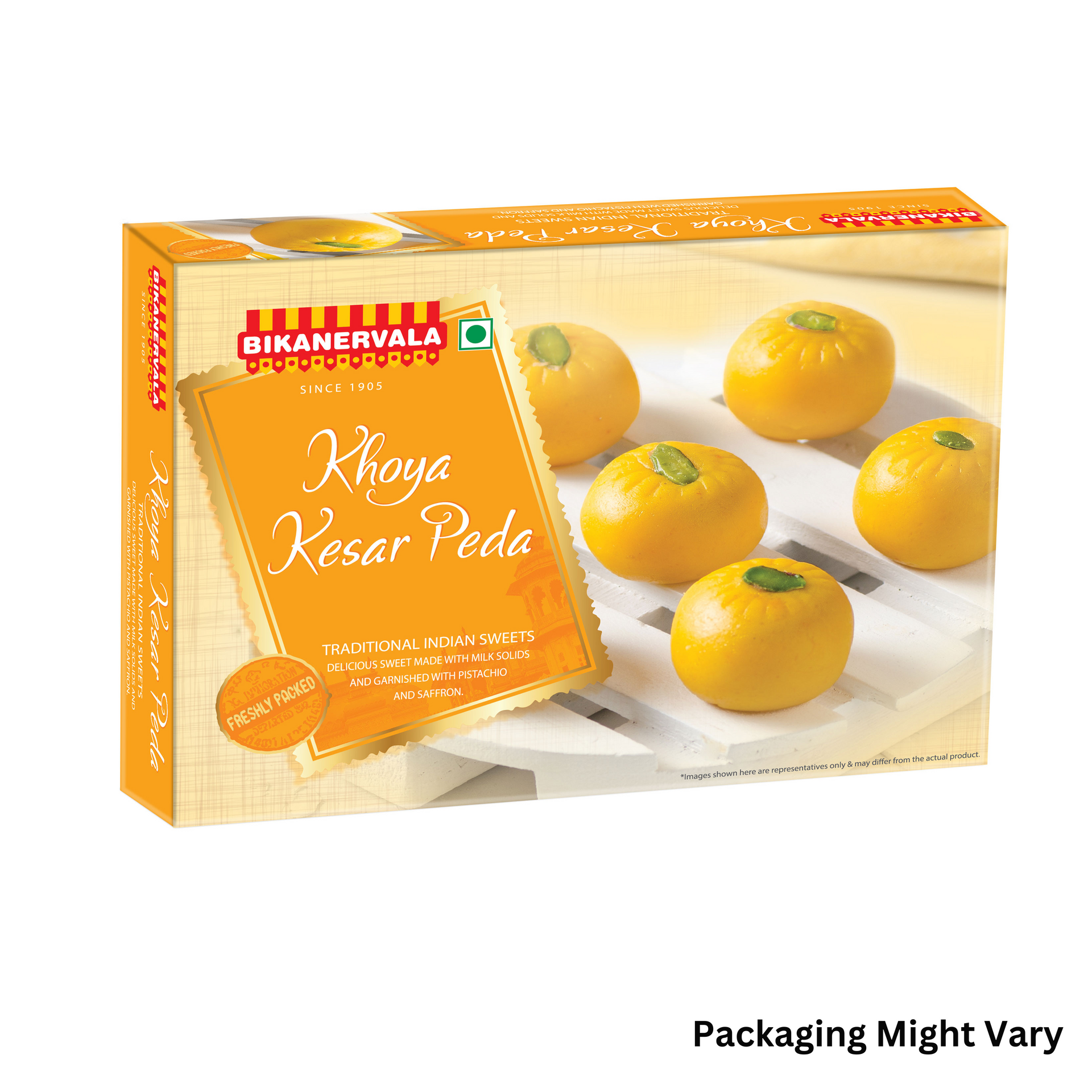This is an image of an advertisement for traditional Indian sweets called "Khoya Kesar Peda." It features a small cardboard box, predominantly white on the top with yellow sides. Inside the box are five yellow, pumpkin-like sweets with green stems, displayed prominently on a white board on a countertop. To the left of the sweets, the brand name "Bikanerwala" is displayed in white text over red and yellow barberpole-like lines. Below the brand name, "Khoya Kesar Peda" is written in white, followed by the phrase "Traditional Indian Sweets" and a note that says "Freshly packed, packaging might vary."